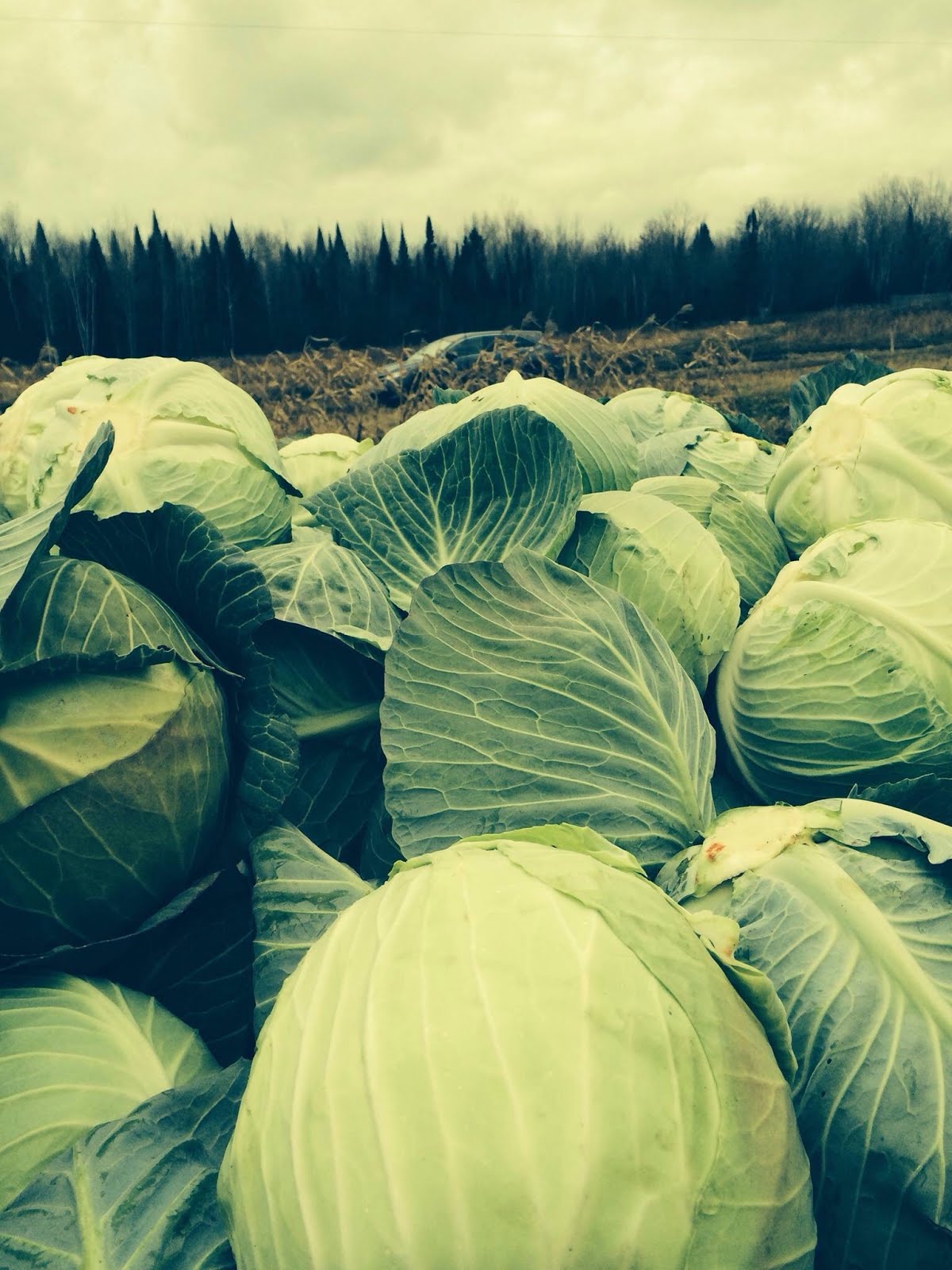The photograph captures a collection of freshly harvested heads of cabbage piled in the foreground, their vibrant green and yellowish hues contrasting against the overall yellowish tint of the image. Each cabbage appears fresh with tightly bound leaves, although a few have slightly disrupted top leaves. The setting is a field or farm, indicated by the visible brown stalks and long grass. In the background, a car is parked, and tall trees line the horizon. The overcast, gray sky gives the scene a muted lighting, enhancing the earthy ambiance.